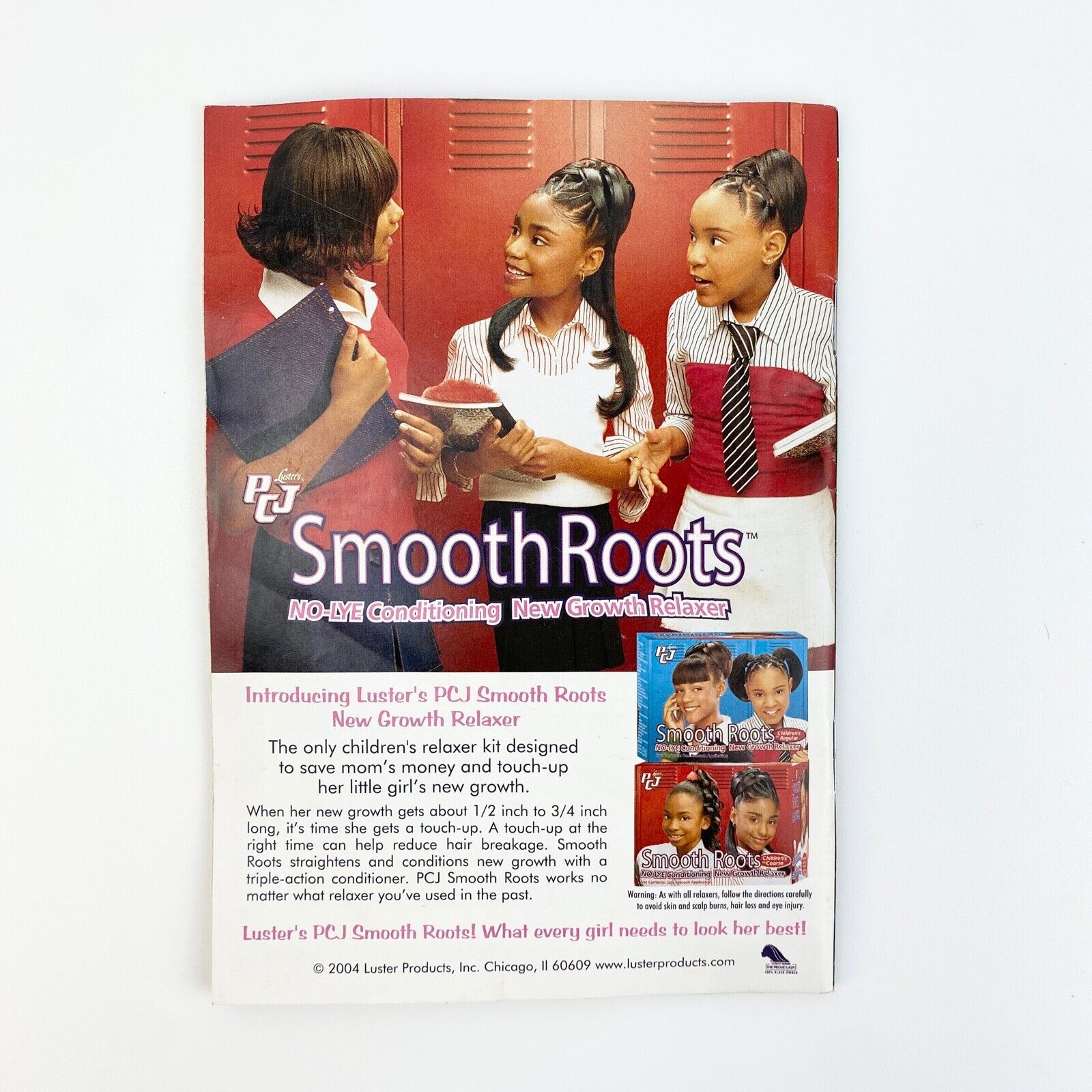This image is a 2004 advertisement by Luster Products Incorporated for the PCJ Smooth Roots No-Lye Conditioning New Growth Relaxer. It features three African American girls standing in front of red lockers in what appears to be a high school setting. The girls are dressed in school uniforms and hold books and notebooks, engaged in conversation. Their hairstyles vary: the girl on the left has a bob that swoops upward at the ends, the girl in the middle has her hair in a half ponytail, and the girl on the right has her hair fully up in a ponytail. The advertisement highlights the product as the only children's relaxer kit designed to save mothers money and effectively touch up new hair growth. The bottom of the advertisement displays two images of the product packaging, emphasizing its benefits and appeal to young girls aiming to look their best.